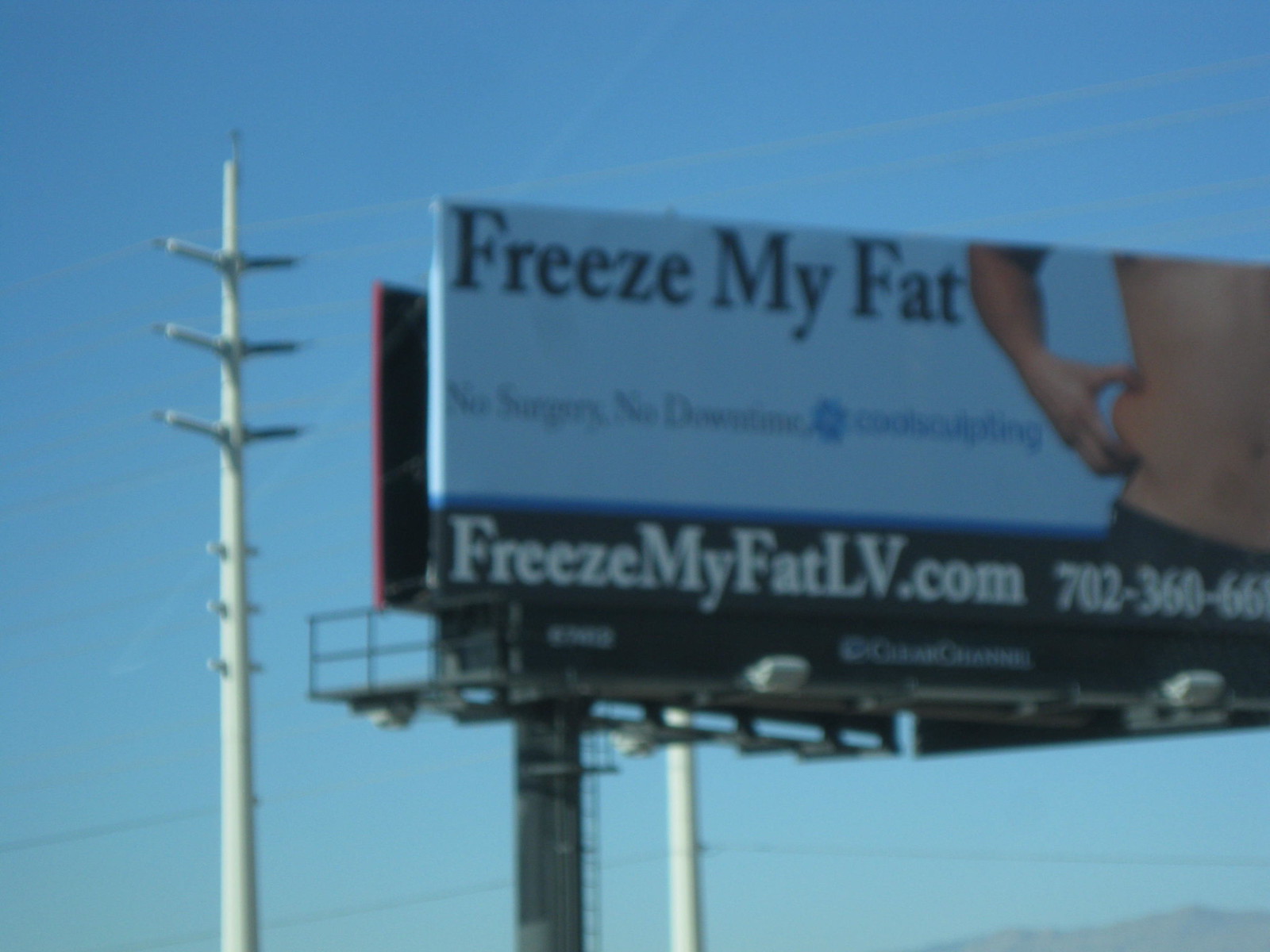The photograph captures a billboard set against a gradient blue sky, transitioning from medium blue at the top to light blue at the bottom. In the background, a power line pole is visible, adding a touch of urban infrastructure to the scene. At the bottom right-hand corner, the top of a hill or mountain range subtly peeks into the frame, providing a hint of natural landscape.

Dominating the middle right portion of the photograph, the billboard advertises a body contouring service. Though not fully within the frame, the text on the billboard clearly displays the words: "Freeze My Fat. No surgery, no downtime, CoolSculpting." A web address is prominently featured as "freezemyfatlv.com," along with a partially visible phone number, showing the digits "702-360-66." The advertisement and its details are sharply rendered, creating a striking contrast against the picturesque sky.